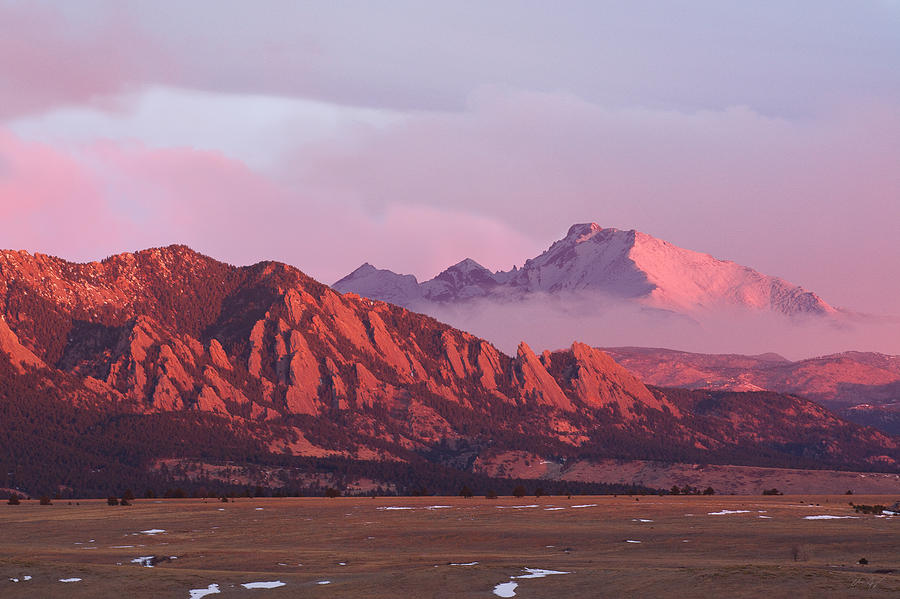This professionally taken landscape photograph showcases a stunning mountain range during sunset. The foreground features a vast, sandy floor interspersed with patches of water, hinting at recent rainfall. The sandy terrain is a greenish-brown, adding depth and contrast to the scene. The primary mountains dominate the midground, cloaked in a mesmerizing reddish, auburn hue with shades of pink, peach, orange, and red. This vivid coloration is further accentuated by the setting sun. Scattered small trees and greenery are visible, clinging to the rugged slopes. In the background, a secondary mountain range appears, its peaks capped with white snow and partially shrouded in fog. The sky above is a gradient of blue, gray, pink, and purple tones, with hazy clouds adding to the ethereal quality of the image. Throughout the scene, there are no people or animals, emphasizing the untouched and tranquil beauty of the natural environment.